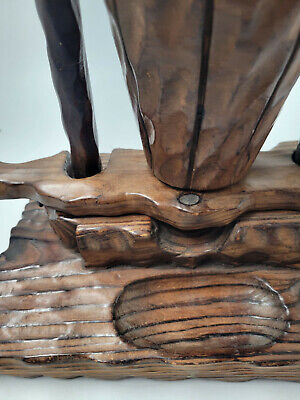The image depicts a detailed close-up of a woodworking piece comprising multiple layers of natural, dark wood, each finished with a shiny varnish that accentuates the wood's rich, brown color and visible grain streaks. The structure features a flat base with a smaller, hollowed-out bowl carved into its center. Stacked atop this base is another wooden piece with a carved lip, followed by a round, branch-like piece attached with a silver nail. On the left side of the base, a thinner, rounder piece of wood extends outward, with a metal rod nearby, possibly serving as a pivot or support. At the very top, there's a vase-shaped, beveled piece suggesting that the design might allow water to flow from the top into the hollowed bowl below. The intricate assembly of wood layers and metal components suggests a functional yet decorative woodworking creation, possibly a stand or a unique artisanal object.